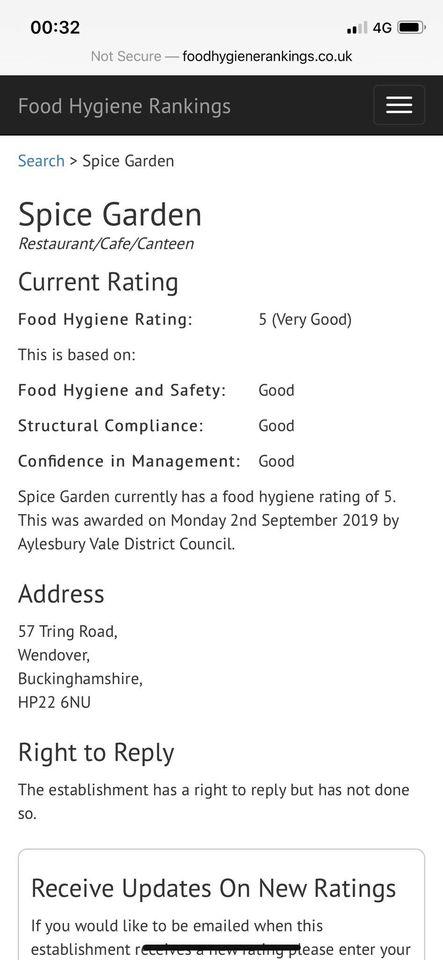This is a detailed screenshot capturing the food hygiene rankings for a restaurant called Spice Garden. The background of the image is predominantly white.

At the very top, a light gray rectangle spans across the width of the screenshot. In the upper left corner, there is a piece of black text reading "0032." To the right, there are icons indicating connectivity bars, followed by "4G," and a battery indicator.

Below this gray rectangle is a URL bar with the text "Not secure - foodhygienerankings.co.uk."

A black rectangle with light gray text follows beneath the URL bar, stating "Food Hygiene Rankings." On the right side of this black rectangle, there are three vertically stacked bars.

Underneath this section, aligned to the left, is a search field reading "Search Spice Garden." Below the search field, the details of the Spice Garden restaurant/café/canteen are presented. Black text specifies "Spice Garden Restaurant/Cafe/Canteen," followed by "Current Rating: Food Hygiene Rating: 5 (Very Good)."

The rating is attributed to several categories:
- Food Hygiene and Safety: Good
- Structural Compliance: Good
- Confidence in Management: Good

A detailed description adds that Spice Garden currently holds a food hygiene rating of 5, awarded on Monday, 2nd September 2019, by Aylesbury Vale District Council.

Further information includes the address:
"57 Tring Road, Wendover, Buckinghamshire, HP22 6NU."

The screenshot also notes the "Right to Reply" stating that the establishment has not yet exercised this right. Lastly, there is an option to "Receive updates on new ratings."